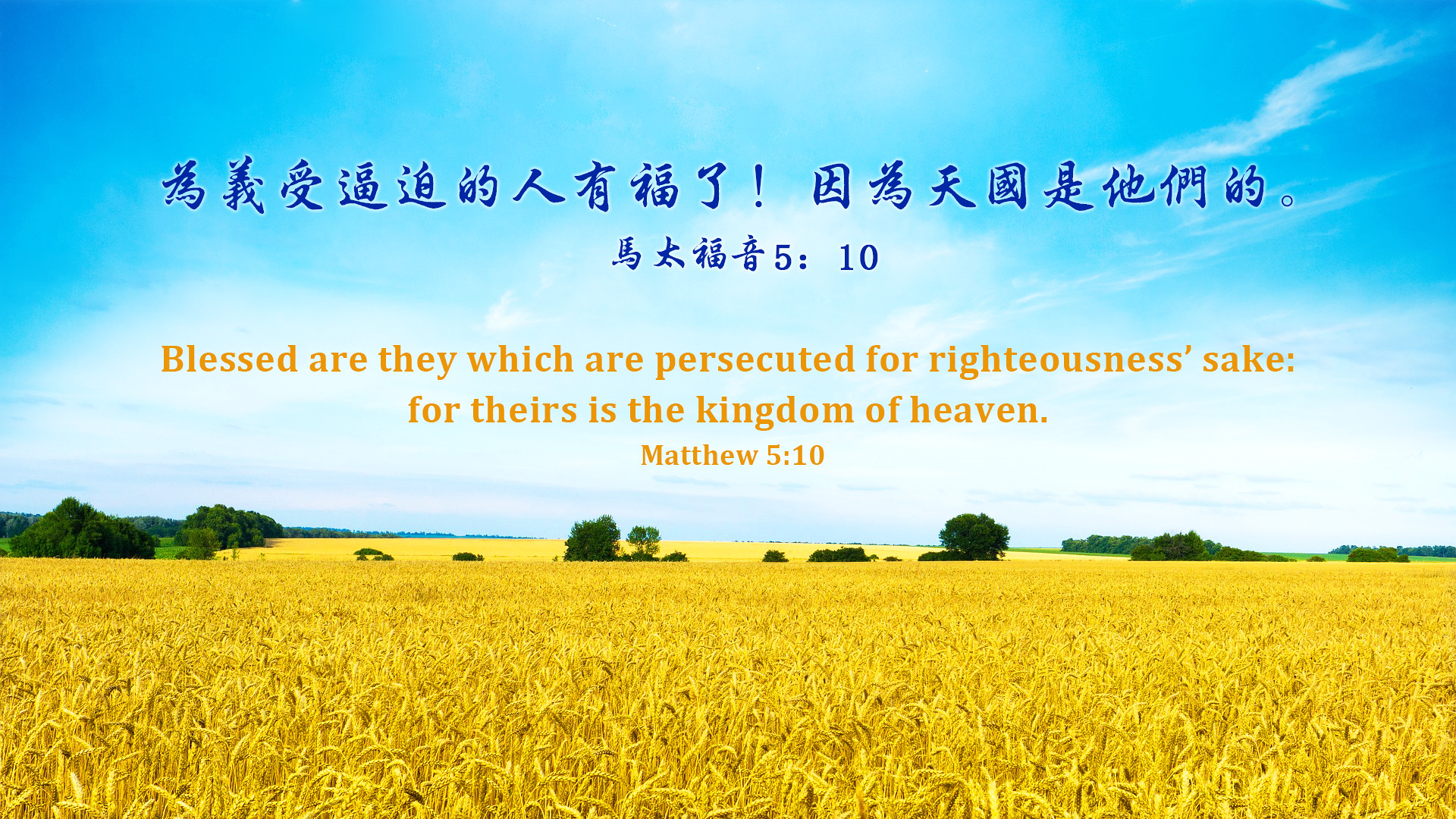The image features an inspirational quote superimposed over a picturesque outdoor scene. The photograph is wider than it is tall, resembling the shape of a high-definition television. The top half of the image displays a light blue sky dotted with multiple white clouds, indicating a sunny day. The horizon is adorned with some distant hills and trees. The bottom half captures endless fields of yellow wheat stretching to the horizon, intermittently punctuated by large trees with lush green leaves on the left and right sides.

The top portion of the text is written in Asian characters, possibly Japanese or Chinese, in blue color. Below this, in yellow text, is the English translation from Matthew 5:10: "Blessed are they which are persecuted for righteousness' sake, for theirs is the kingdom of heaven." The serene landscape paired with this uplifting scripture provides a poignant visual and spiritual experience.